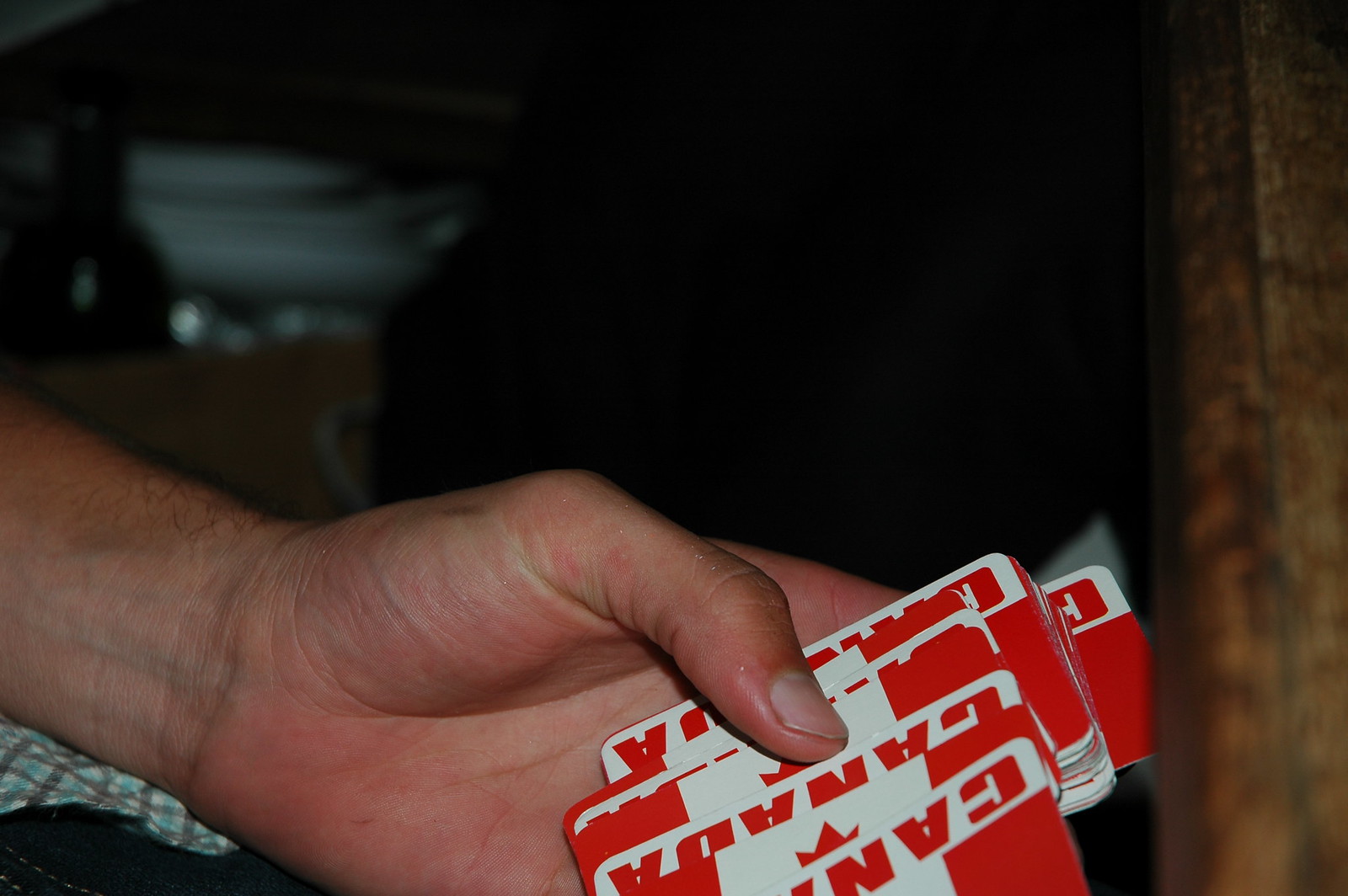This horizontal color photograph captures a person's hand holding a deck of red and white cards with the word "Canada" prominently displayed on the back. The setting is enveloped in darkness, making it indistinguishable whether the scene is indoors or outside. A soft, indirect light—possibly from a flashlight or lamp—illuminates the hand from above, casting gentle shadows. The hand, appearing to belong to a male, reveals a slightly bitten thumbnail and some arm hair. Beneath the wrist, there's a hint of checkered fabric, suggesting the person might be wearing a checkered shirt. The cards are not turned over, leaving the faces hidden and the card types—such as hearts or spades—unknown.